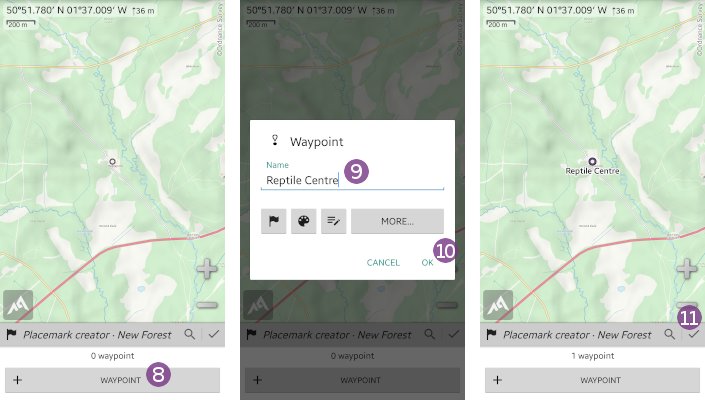This image is a composite screenshot taken on a phone, displaying three different segments side by side, likely from a mapping application. 

1. **First Segment**: This segment portrays a map interface with a green and white backdrop, featuring a small circle at the center. At the top of this section, coordinates are displayed: "5051.780 North" and "137.009 West," along with an elevation reading of "36 m". Towards the bottom, text reads "Placement Creator - New Forest Waypoint," and prominently below is "WAYPOINT" in capital letters followed by the number "8".

2. **Middle Segment**: The middle screenshot overlays a white box onto the map background similar to the first segment. Inside this box, the word "Waypoint" is followed by a designated name: "Reptile Center," associated with the number "9". This section includes icons for a flag, paint, and notes, along with a "More" button. Below these, there are "Cancel" and "Okay" buttons, with the number "10" positioned beside the "Okay" button.

3. **Third Segment**: This part closely resembles the first segment, retaining the green and white map background and centralized circle. The main difference here is that instead of displaying the number "8" like in the first segment, it shows a "purple circle" with the number "11" in white at the bottom right-hand corner.

Each segment presents a different stage or feature of what seems to be a waypoint placement or creation on the mapping application.